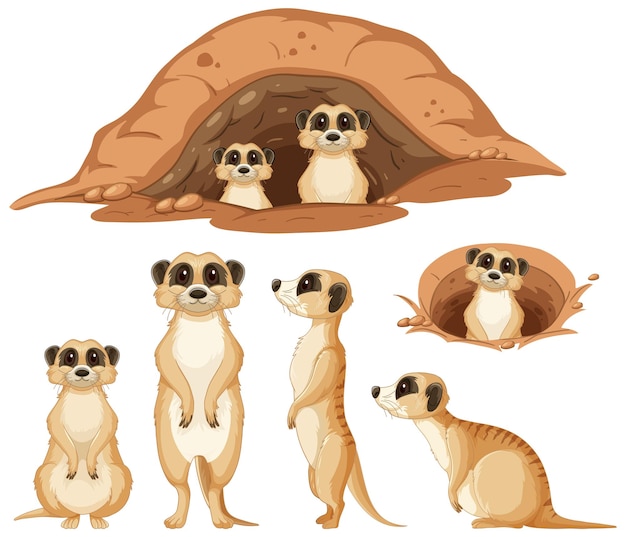This illustration features a playful and cartoonish depiction of seven meerkats set against a white background. At the very top, there is a rounded brown hole with dirt around it, from which two meerkats are peeking out—the one on the left is shorter than the one on the right. Both meerkats have tan bodies with lighter tan chests, brown eyes with large black pupils, dark brown ears with black insides, and similar facial expressions. On the right middle side of the image, there is another brown, dirt-rimmed hole with a single meerkat peering out, showcasing only the top half of its body.

At the bottom, there are four meerkats with distinct postures. The first one on the left is squatting down. The second meerkat, next to it, stands tall with its legs fully extended. The third meerkat faces the left in a crouched position, revealing brown stripes on its back. The fourth meerkat, also facing left, is sitting on its rear. Despite their different stances, all meerkats share the same facial features, characterized by gray markings around the eyes, gray ears, and brown eyes, which give them a cohesive look.